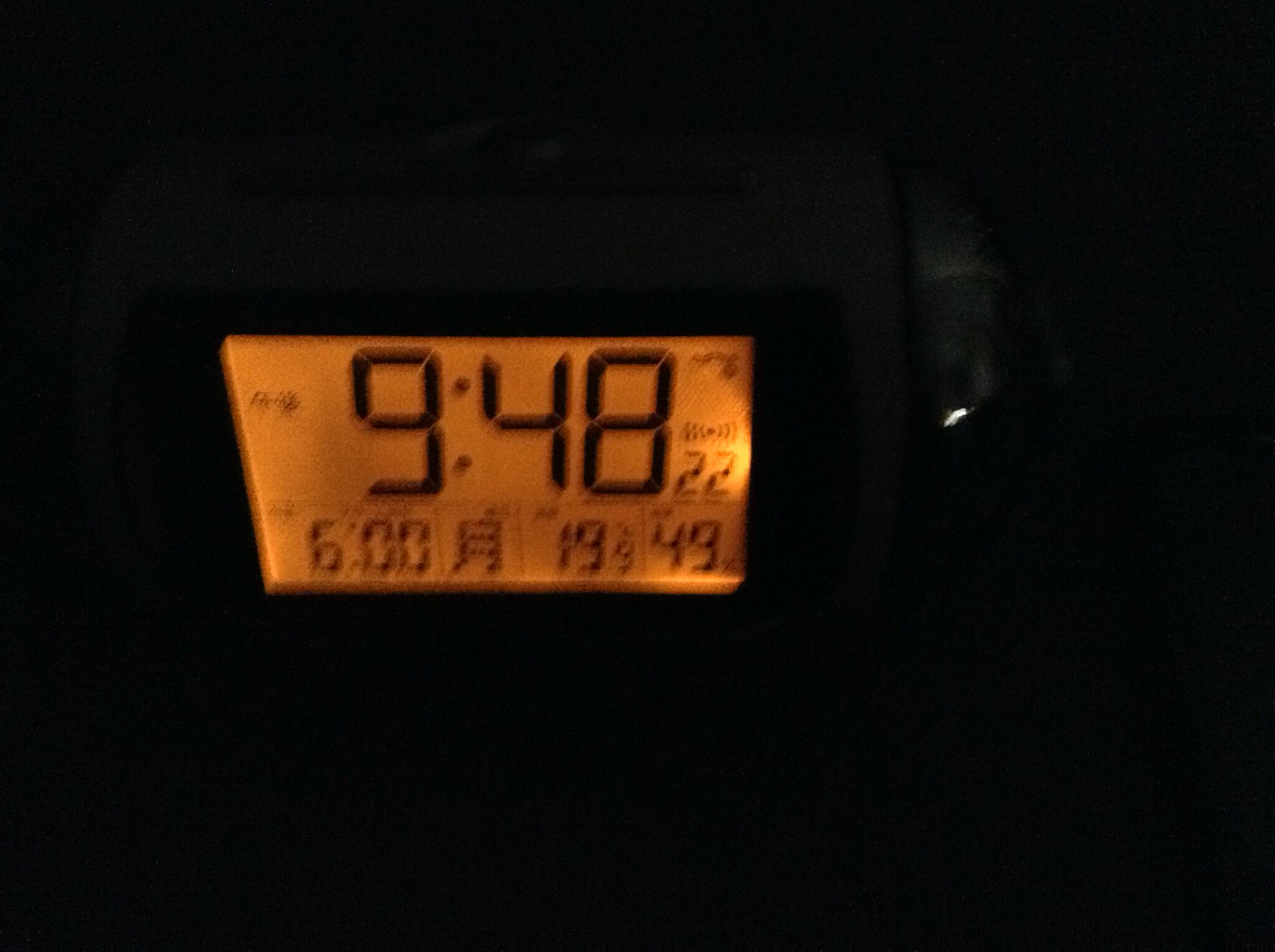In this nighttime photograph, the surrounding environment is shrouded in darkness, with the exception of the illuminated face of a digital clock, which casts a soft, yellowish light. The clock prominently displays the time as 9:48:22. Below this, additional numbers are visible: "6:00," "19:09," and "49," which might indicate secondary information such as an alarm setting or date. In the far background, there is a faintly lit object that hints at another light source or item in the room, adding a subtle layer of mystery to the scene. The overall composition captures the ethereal quality of light piercing through an otherwise pitch-black space, highlighting the detailed precision of the clock's display.